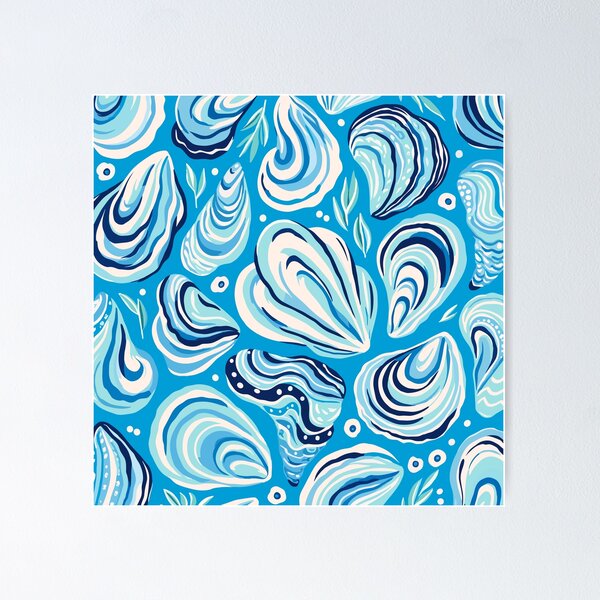The image is a square print featuring a watercolor painting set against a light blue to turquoise background. The central design depicts an array of clam-like shells in varying shades of blue, from dark to very light, interspersed with white. These shells appear in multiple sizes and orientations, creating an intricate, almost floating pattern. Scattered among the shells are delicate details such as small, light green leaves, round dots, and bubble-like circles, some resembling eyes with white and light blue pupils. The overall aesthetic is a vibrant and dynamic composition with no defined outlines, offering a mesmerizing mix of shapes and colors. The print is framed against an off-white background, adding a subtle contrast that enhances the artwork’s vividness.